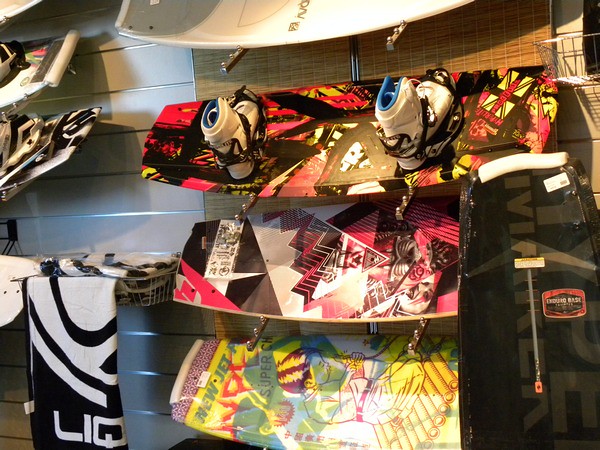The image depicts a retail shop specializing in snowboarding equipment. Numerous snowboards are uniformly displayed on wall-mounted metal racks featuring ball stoppers. The snowboards rest angled uniformly on the third ball of each rack, and the overall presentation is neatly aligned. The backdrop consists of a gray wall segmented into board-width panels, accompanied by wooden window shades extending almost across the entire wall width. To the left, a small wall-mounted basket holds a folded black and white towel. Snowshoes, also white, adorn a multicolored snowboard decorated with red, black, and yellow lines. Visually engaging, the snowboards exhibit diverse designs including white with black markings, a vibrant mix of pink, yellow, and red, and striking patterns of zigzags and stripes. On the bottom row, a yellow snowboard features blue and red writing, and a black fabric bag for snowboard equipment is positioned in the bottom right corner. The overall scene is a visually elaborate display of snowboarding gear within a sophisticated retail environment.